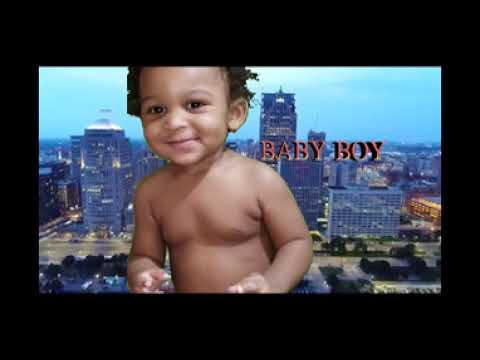The image features a baby boy, approximately three to four months old, smiling and standing with his right hand outstretched, his fuzzy hair and darker skin prominent against the backdrop of a modern cityscape. Encased in a black frame that is wider at the top and bottom than on the sides, the picture captures the boy towering over a variety of tall, bluish skyscrapers and buildings, creating a fantastical "Godzilla-like" effect. To the right of the boy, the words "Baby Boy" are printed in red. The city's background is a mix of light blue sky and a lit-up cityscape with a double-sided highway, neighborhoods, and a vertical yellow or gold-ish rectangular building standing out in the center. The daytime scene is lively, with a park and trees in the foreground of the glass office buildings, enhancing the juxtaposition between the towering toddler and the urban environment.